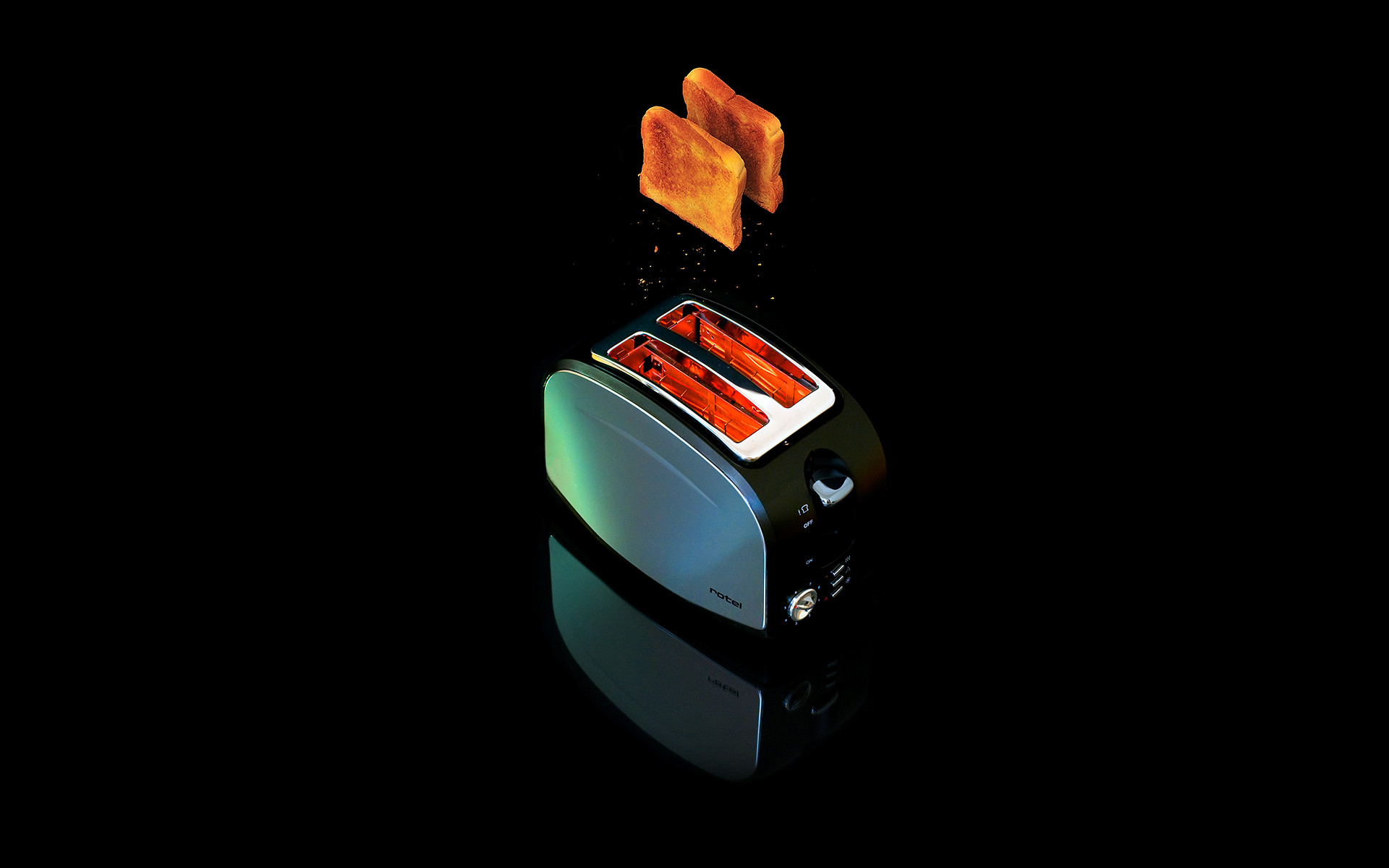The image depicts a sleek, modern toaster with a silver face, black sides, and silver buttons and knobs. Its heating elements are visibly glowing, indicating the toaster is in use. Suspended about a foot above the toaster are two slices of toast, captured mid-air as they seemingly pop up, with some crumbs spilling off due to the sudden motion. The toast is well-done, sporting a mix of light brown and darker, scorched sections. The backdrop is a plain black, with a glossy surface that reflects both the toaster and the hovering slices, adding a dramatic contrast to the scene.